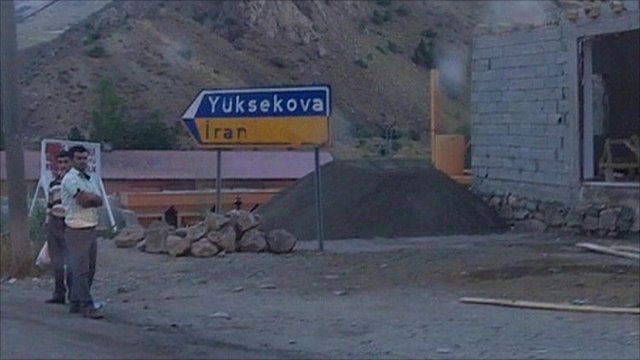In the foreground of an old photograph, likely taken at night, two men stand on the left side of a street near a directional sign marked "Yuksekova, Iran" that is propped up by boulders and gravel. The sign features a blue and yellow color scheme with an arrow pointing towards Iran. Both men are dressed in slacks and shoes. The man at the front, facing the camera with a serious expression, wears a short-sleeve button-up white shirt and gray dress pants, his arms crossed. Beside him, partially behind and shorter, the second man is slightly turned away, in a striped tan and white long-sleeve shirt, holding a plastic grocery bag. The backdrop includes a large mountain and a whitewashed brick building with an open doorway to the far right. The photograph’s color scheme emphasizes bright whites and browns, with a stretch of road visible in the left corner running up the hillside.